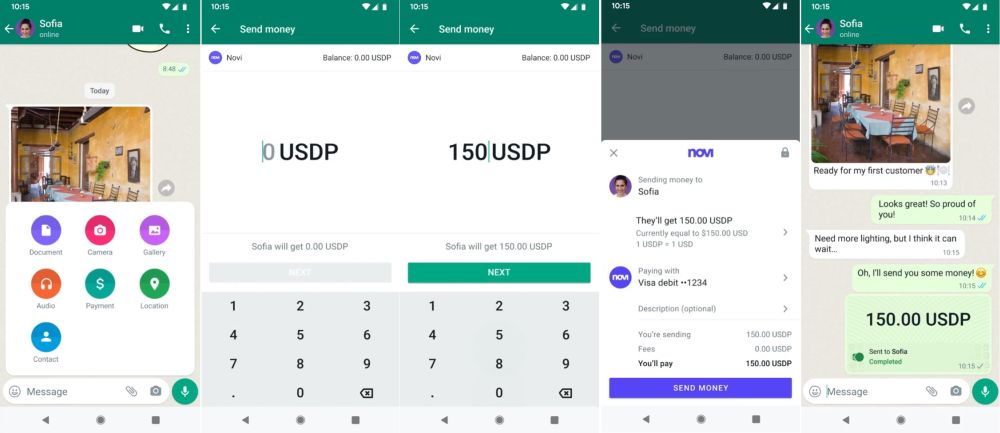This image comprises five different screenshots from a cell phone, depicting a series of actions and interactions related to a chat and money transfer. 

**First Screen (Leftmost):**
- The interface exhibits a green bar at the top featuring a photo of a woman named 'Sophia' in white lettering.
- On the right side of this bar, there are icons for initiating a video call (camera), a voice call (phone), and accessing additional settings (three dots).
- The chat interface below offers various action buttons: Documents, Camera, Gallery, Audio, Payment, Location, and Contacts.

**Second Screen:**
- The green bar now reads "Send Money." The screen prominently displays "0 USDP," indicating an initial state for a money transfer.

**Third Screen:**
- Similar to the previous screen but now showing "150 USDP," suggesting an entered amount ready for transfer.

**Fourth Screen:**
- This is a confirmation page affirming the transfer details:
  - The message reads: "Sending money to Sophia. They'll get 150 USDP."
  - The payer's card details are shown along with a breakdown of the transfer:
    - Sending Amount: 150 USDP
    - Fees: 0 USDP
    - Total to be paid: 150 USDP 

**Fifth Screen (Rightmost):**
- The chat interface with Sophia is back on display. The conversation reads:
  - From the user: "Ready for my first customer. Looks great. So proud of you. Needs more lighting, but I think it can wait."
  - From Sophia: "Oh, I'll send you some money."
- It indicates that Sophia has sent 150 USDP to the user, with the user needing to click to accept this transfer.

This detailed caption provides a comprehensive overview of the sequence and context presented in the image.